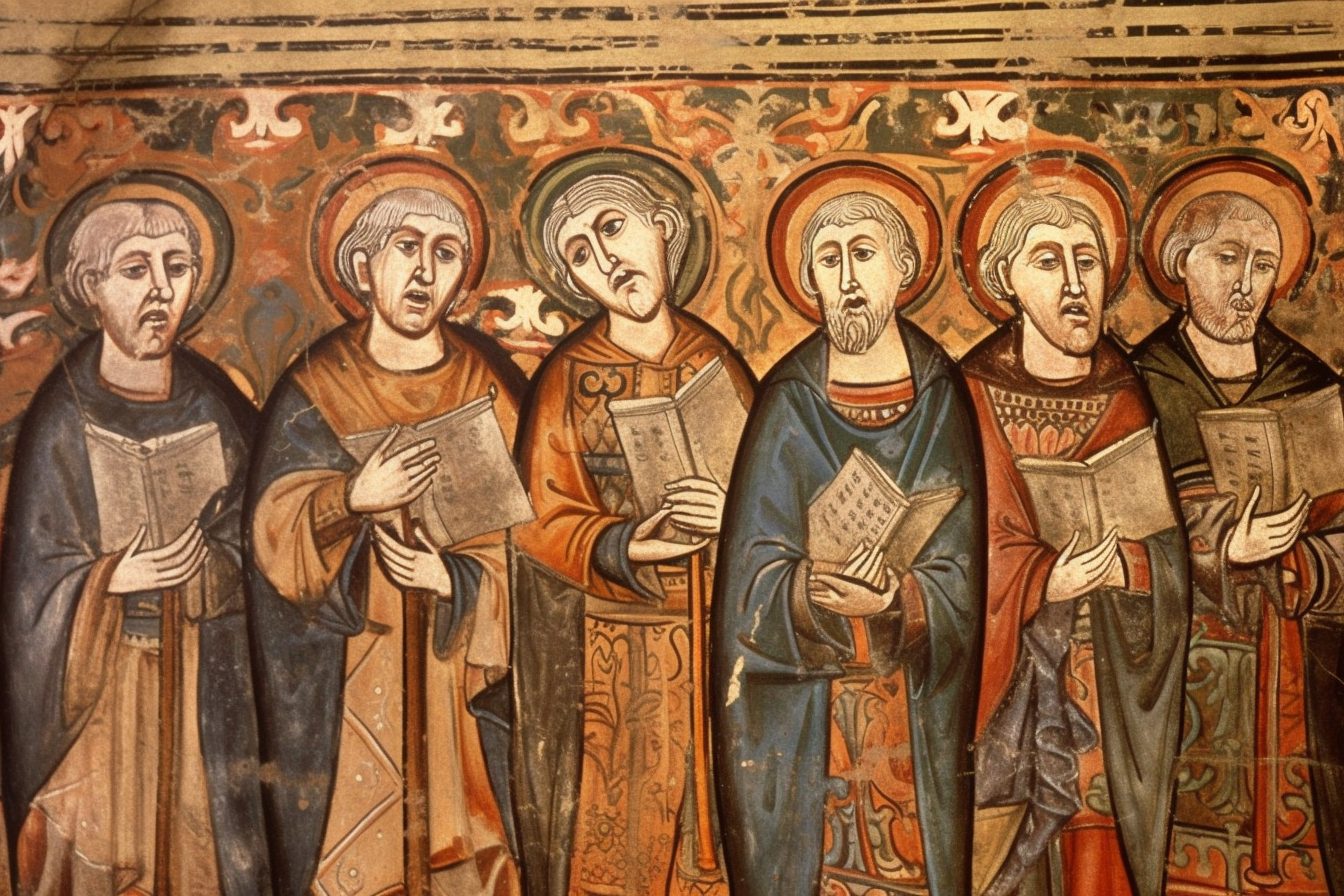The image is a detailed and melancholic painting that likely adorns the walls of an old church, characterized by its rich, warm palette of oranges, reds, tans, and interspersed hues of green, blue, beige, and dark blue. It depicts six solemn men who appear to be religious figures such as priests, monks, or possibly saints, indicated by the circular halos around their heads. Clad in orange and black robes, they stand in close proximity, each holding a booklet that resembles a singing book or hymnal. Their expressions are uniformly mournful, with heads tilted or bowed, and mouths in various states of being open or pursed, suggesting they might be engaged in singing or prayer. The background is adorned with subtle, complementary designs, seamlessly blending with the overall color scheme and enhancing the sense of antique religious iconography.